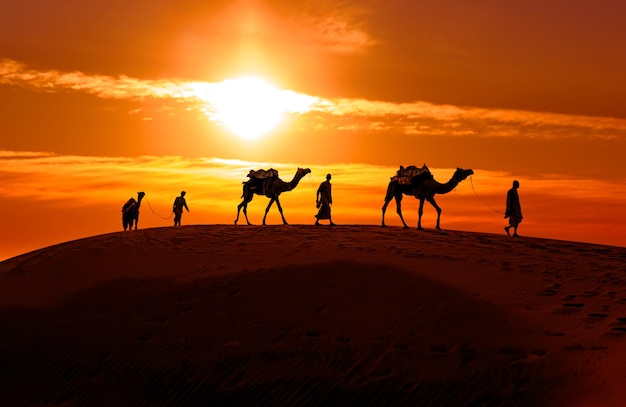In the image, a breathtaking desert landscape unfolds under a mesmerizing, vividly orange and yellow sunset sky, radiating such brilliance it nearly hurts the eyes. Dominating the scene is a vast sand dune, accentuated by its distinctive brownish-orange hue, transformed by the intense sunlight. Silhouetted against this glowing backdrop, three camels and their three handlers traverse in single file, each man leading a camel by a rope. The figures appear as dark shapes due to the low angle of the sun, which obscures their details and emphasizes their outlines. One man near the front descends the dune, the second follows slightly behind, and the third, further back, just crests the ridge, highlighting the perspective and scale of the scene. The overall composition marvelously captures the serene yet rugged beauty of the desert at dusk, with the camels and men etched dramatically against the vibrant, setting sun.